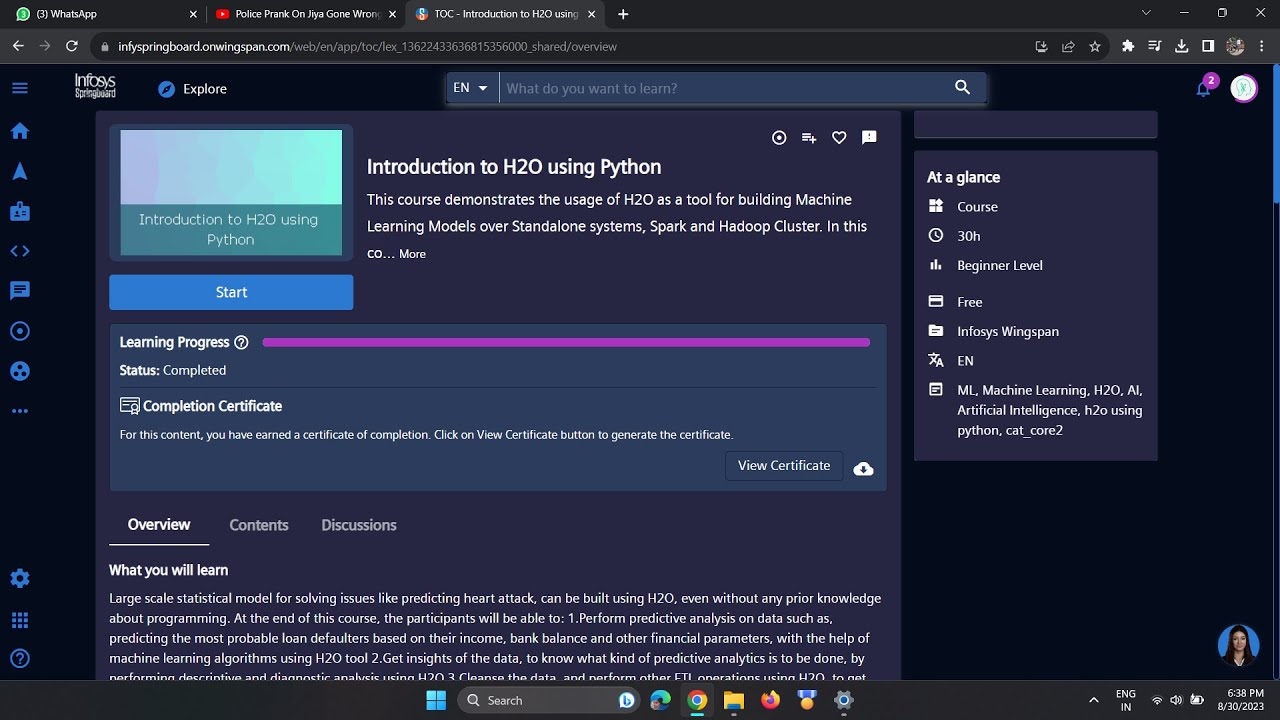This image is a cropped screenshot of a desktop browser displaying three open tabs. The focus is on the third tab, which is an Infosys website specifically on a blog titled "Introduction to H2O using Python," found within the learning section of the site. 

The browser has a dark theme with a black background. Along the far left side, a thin vertical blue panel features several icons: at the top is a home icon, further down is a radioactive symbol, and at the bottom are a cogwheel (settings) and a question mark (help).

At the top of the page, the Infosys logo is prominently displayed, adjacent to which is an "Explore" button. Toward the center right is a search box with a drop-down menu set to "EN" for English.

The main content area features a large black box on the left where a photo thumbnail is visible along with a blue "Start" button underneath it. On the right, the heading "Introduction to H2O using Python" is displayed with a brief description below it.

Further down, a dark blue rectangular section labeled "Learning Progress" is shown, featuring a purple status bar. The text below indicates "Status: Completed," along with options to view or download the completion certificate. 

At the bottom of the screen, navigation tabs read "Overview," "Contents," and "Course Discussions," with "Overview" currently selected and underlined in white.